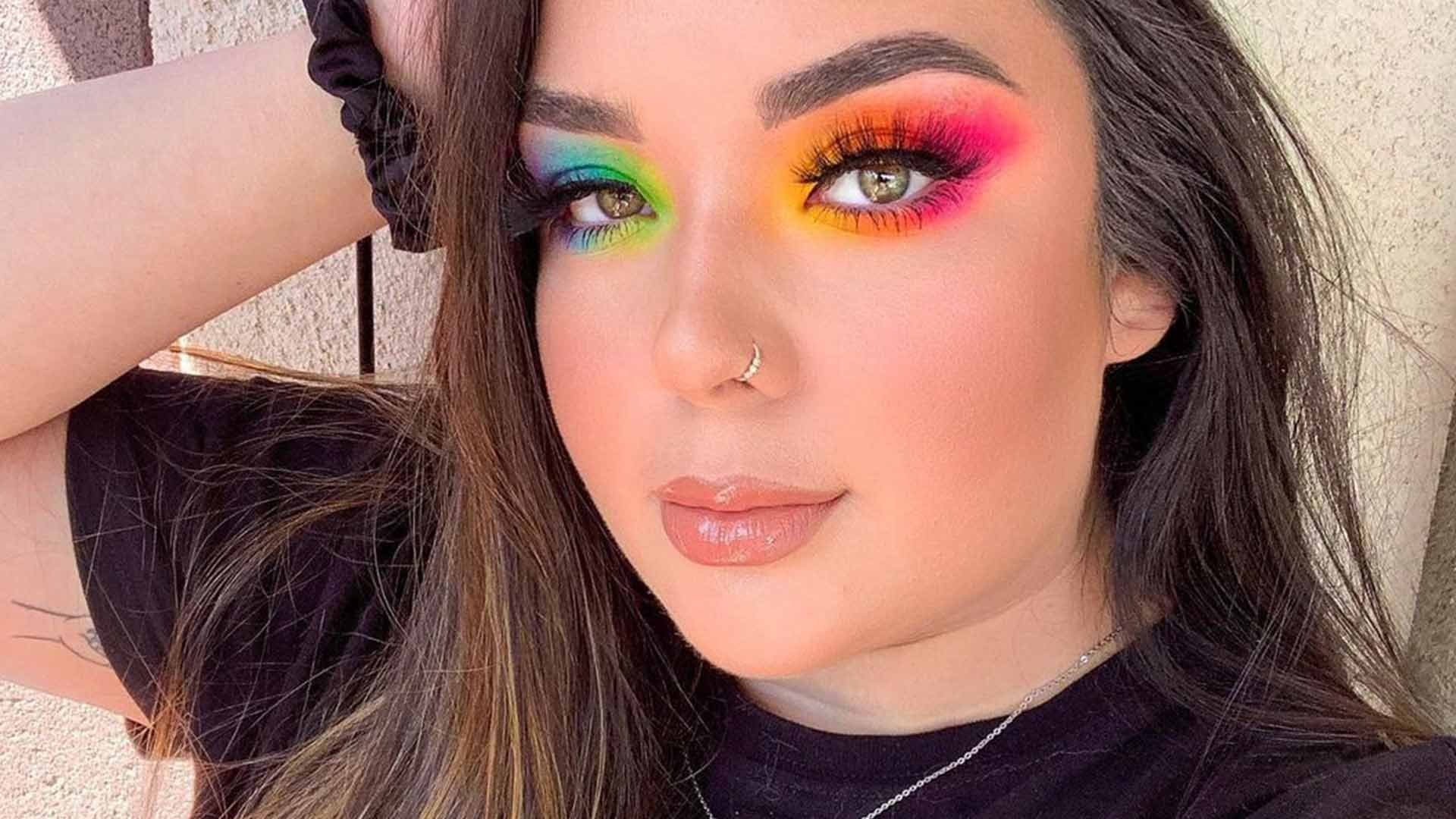In this close-up image, we see a young woman, likely in her mid to late 20s, with a striking and well-crafted appearance. Her face is visible from her neck upwards, with her right arm angled up and resting on her head, and a hair scrunchie adorning her wrist. Her complexion is fair, with black, meticulously manicured, and possibly microbladed eyebrows. She wears vibrant, multicolored eyeshadow: her right eye features a blend of blue, purple, and yellow, while her left eye showcases orange and pink hues. Her thick, elegantly styled, long hair is parted, with the right side appearing brown and the left side black, interspersed with hints of gray.

She has a clear, natural skin tone, enhanced by flawless makeup, and wears a gold nose ring with diamonds. Her lips are noticeably full and polished. She sports a thin silver chain around her neck and a short-sleeved black shirt. On her right bicep, there's a tattoo of a hand. The background suggests she is standing in front of a concrete wall, adding an urban, edgy feel to the portrait.